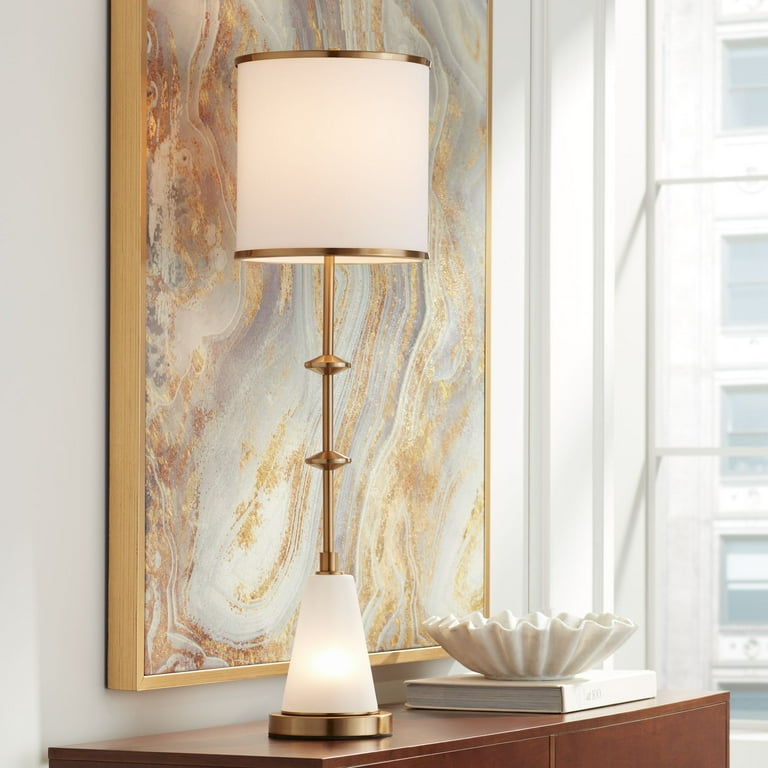This photograph, taken indoors and likely inside an apartment, features a brown wooden cabinet prominently positioned at the center bottom of the frame. On the cabinet rests a large hardcover book, atop which sits a white ceramic dish shaped like a clamshell. Adjacent to these items, on the left side, stands an elegant lamp with a cylindrical white lampshade bordered with gold rims. The lamp has a golden pole with two ridges and is anchored by a conical white base on a round gold stand. Behind the cabinet, the wall is adorned with an expansive abstract painting that extends beyond the frame, showcasing gold and silver hues, and is set against white walls. To the right of the cabinet, a window with a white frame reveals a view of another white building dotted with a row of windows, emphasizing the indoor setting possibly within a high-rise apartment. The color palette in the image includes shades of brown, white, gold, gray, and beige, creating a harmonious and sophisticated atmosphere.